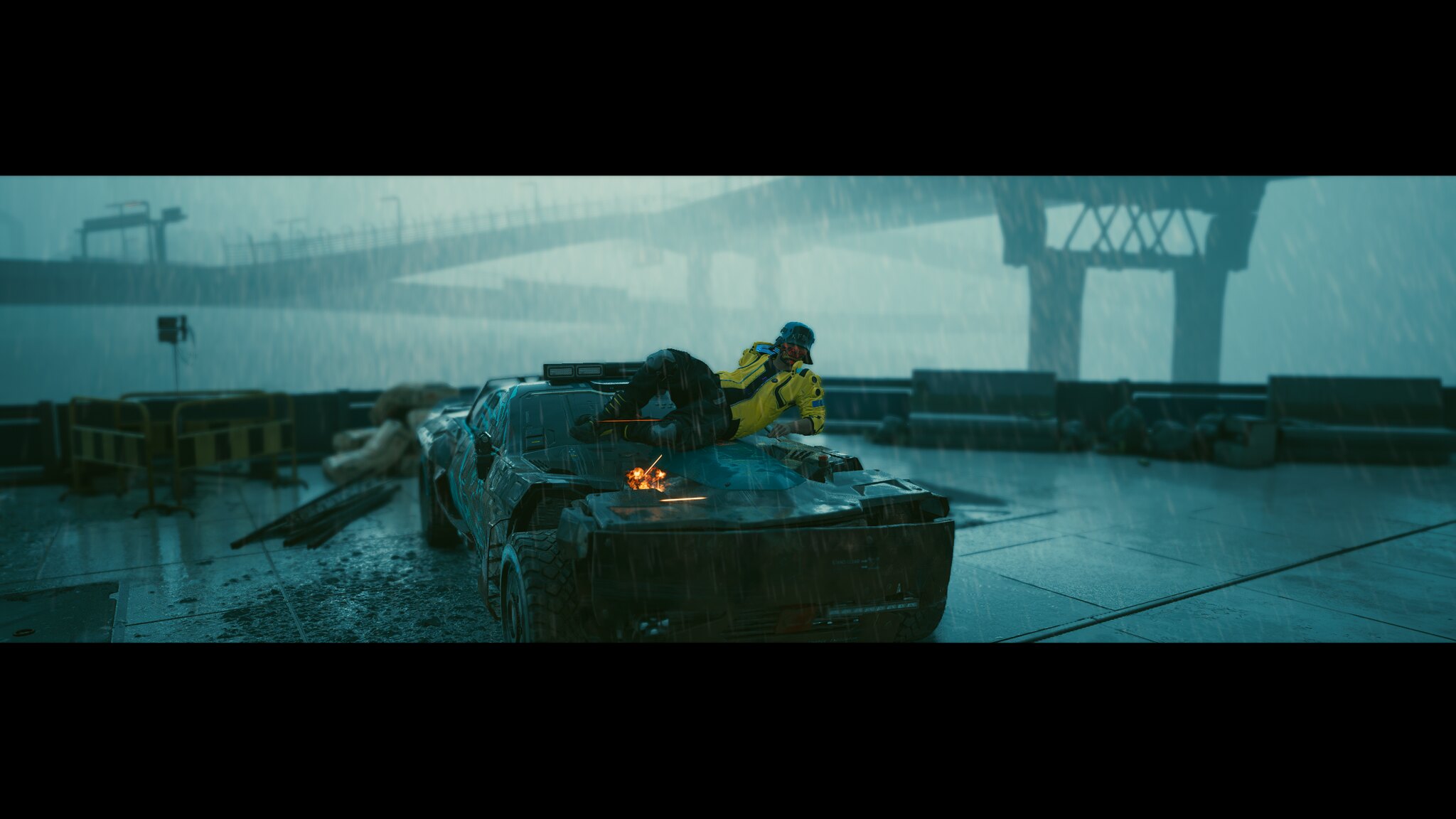In this bluish-tinted, horizontally-framed screenshot from a video game, the scene captures a rainy, foggy environment filled with concrete structures and an intricate network of bridge towers and walkways extending into the distance. In the foreground, a beat-up sports car, likely dark in color—black or possibly a worn greenish-gray—rests angled on a large, tiled platform with rugged tires. The car's front end appears to have sustained significant damage, with smashed headlights, a large gash above the front left tire where the fender would be, and visible sparks. Laying clumsily across the hood and partially onto the windshield of the car is a humanoid figure dressed in dark pants, a yellow long-sleeve jacket, and a backward baseball cap. This figure supports themselves with their arms, adding to the sense of chaos and disarray. The platform is surrounded by traffic barriers, including yellow and black-striped ones, and possibly railings, contributing to the scene's overall cluttered and rundown appearance.